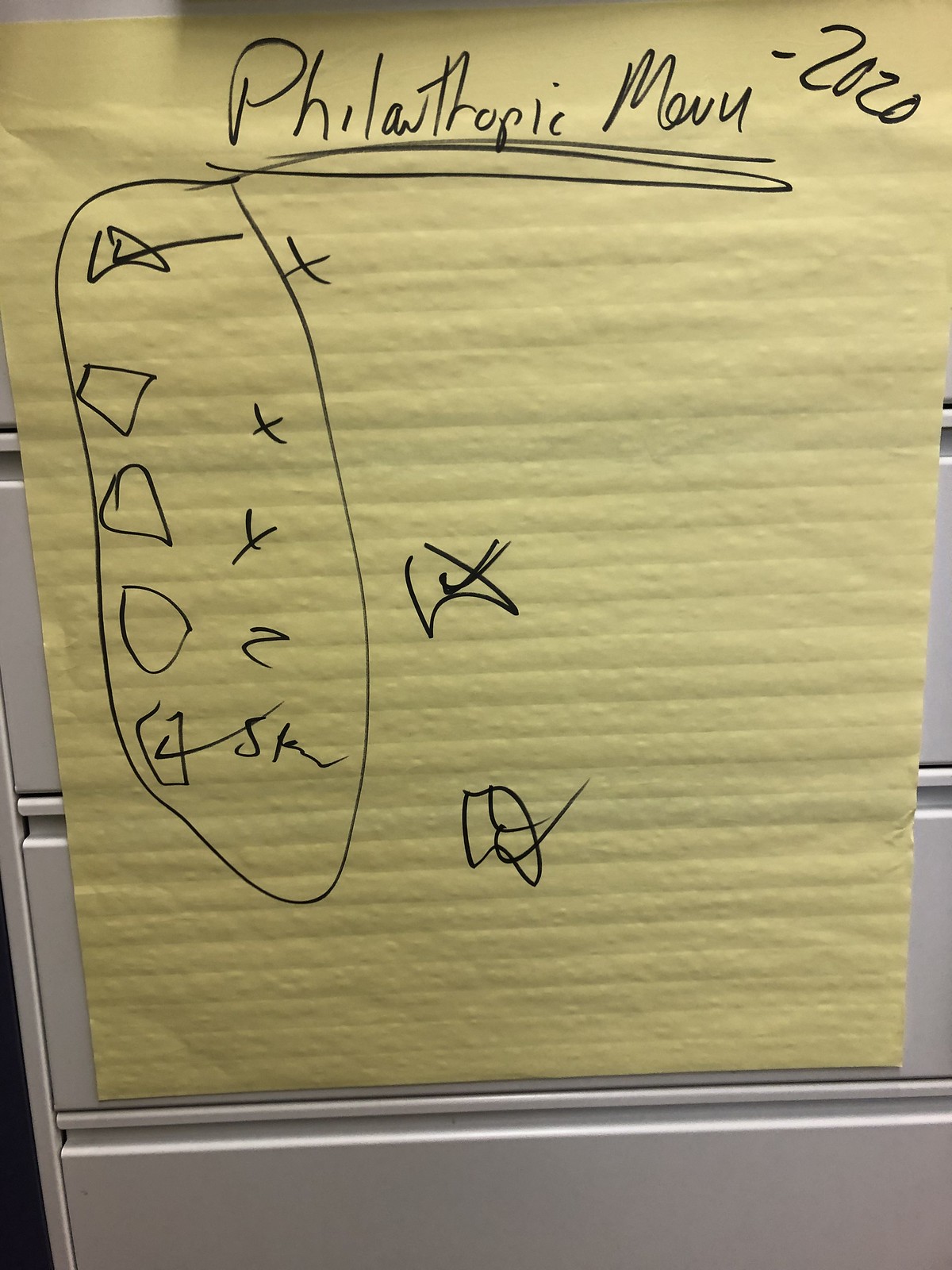In a brightly lit photograph, a thin piece of yellow presentation paper with a sticky top is affixed onto a tall dresser. The paper, illuminated under the abundant light, casts subtle shadows towards the top, possibly from an out-of-focus shelf above. Written with a black Sharpie in messy, hard-to-read handwriting, the paper displays the title "Philanthropic Movie 2020" underlined three times. Below the title, an oval encircles multiple checkmarks and X marks, with several boxes marked and initialed, alongside two additional boxes haphazardly checked. The overall cluttered and disorganized writing captures a snapshot of an evolving project checklist.